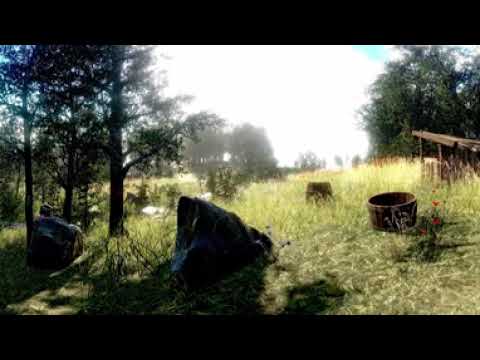The image depicts a pixelated, low-resolution outdoor scene that resembles a vintage video game. Dominating the immediate foreground is a grassy field with overgrown grass about two to three feet tall, some of which have shoots at the top. In the center stands a waist-height boulder, accentuated by its triangular shape and flanked by another square boulder approximately ten feet away from the camera. To the left side of the frame, a cluster of trees provides shade, creating a somewhat sheltered ambiance, while the right side features a little bush adorned with four lonely red flowers. Adjacent to it is a rustic wooden tub or barrel, suggesting an old-fashioned, utilitarian purpose.

Further to the right, a wooden beam emerges, perhaps part of a small canopy or porch-like structure, with grass growing beneath it. Tall, bushy trees extend from the top right corner, their green leaves contrasting with the bright white sky, indicative of sunlight piercing through. A closer inspection reveals shadows towards the bottom portion of the image, hinting at additional trees and possibly a tractor at the distant horizon. The entirety of the scene, from the grassy field to the scattered artifacts and natural elements, captures a serene yet slightly nostalgic woodland setting.